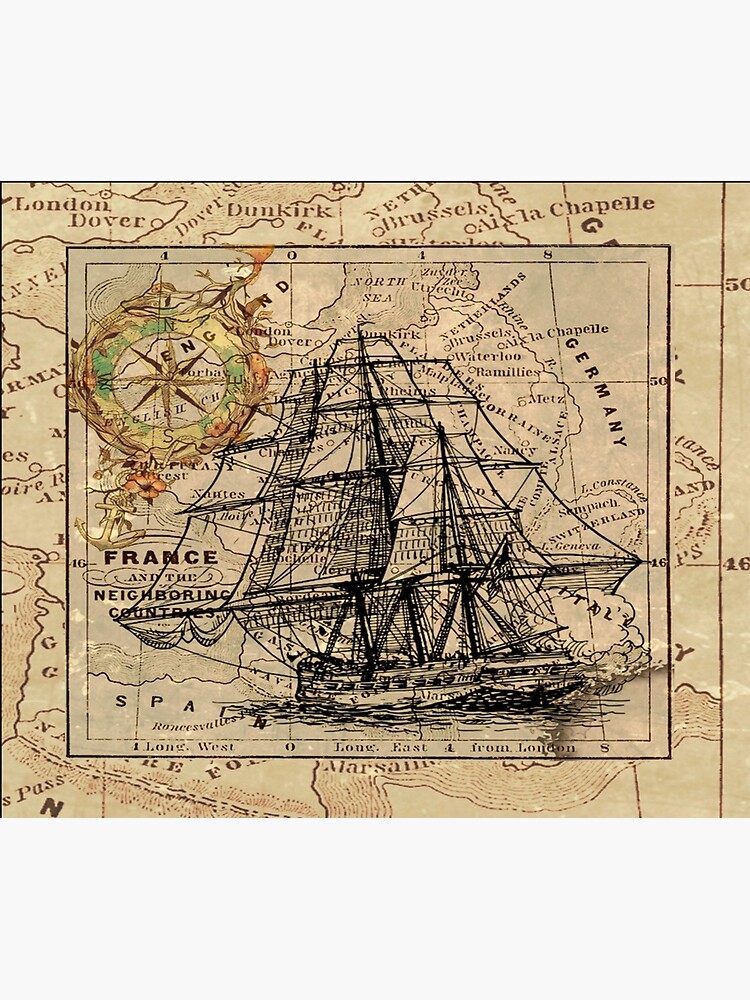The image depicts a detailed and intricate vintage map of Central Europe with a prominent sepia tone, printed on grey-colored paper. At the heart of the composition, a detailed illustration of a boat with large sails is situated directly in the middle, navigating toward the right. Surrounding the boat, the map showcases numerous important regions and cities including Germany, France, Spain, England, Italy, Switzerland, Geneva, Waterloo, and the Netherlands. Key locations such as Dunkirk, London, Dover, and Brussels are also clearly marked. The map features geographical details like land markings and degrees on the borders. Additionally, there is an inset box within the main image depicting a compass in the top left corner, along with maritime elements such as an anchor design and directional pins. The overall setting hints at this being an artistic creation, finely blending cartography and nautical themes in a historical context.